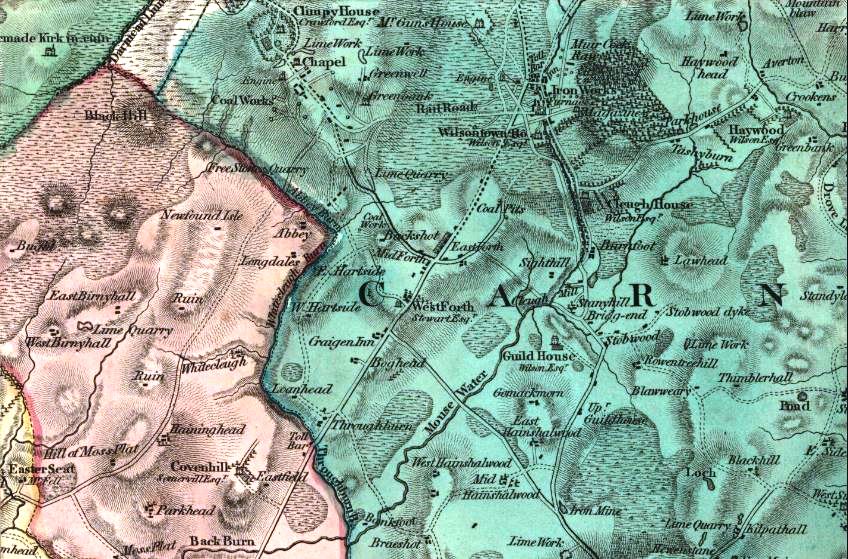This image captures a detailed map divided into distinct colored districts. The left side of the map features a yellow district at the bottom, transitioning to a red-pink district that dominates the majority of the left side. Key locations within the pink district include "Newfound Isle," "Ruin," "Lamb Quarry," and smaller towns like "Cabin Built" and "Backburn." Towards the center, the map shifts to a greenish-teal district on the right-hand side, which includes labels for "Guildhouse," "Thimber Hall," "Pond," "Haywood Head," and "Climb Bee House." The blue-green area prominently features the word "Carn" written in large black letters across its center. The map includes topographical sketches, rivers, and roads depicted with dotted and straight lines. The entire image has a two-tone color scheme with black and gray writing for all labels and landmarks, giving it a distinct, digital, and zoomed-in appearance.